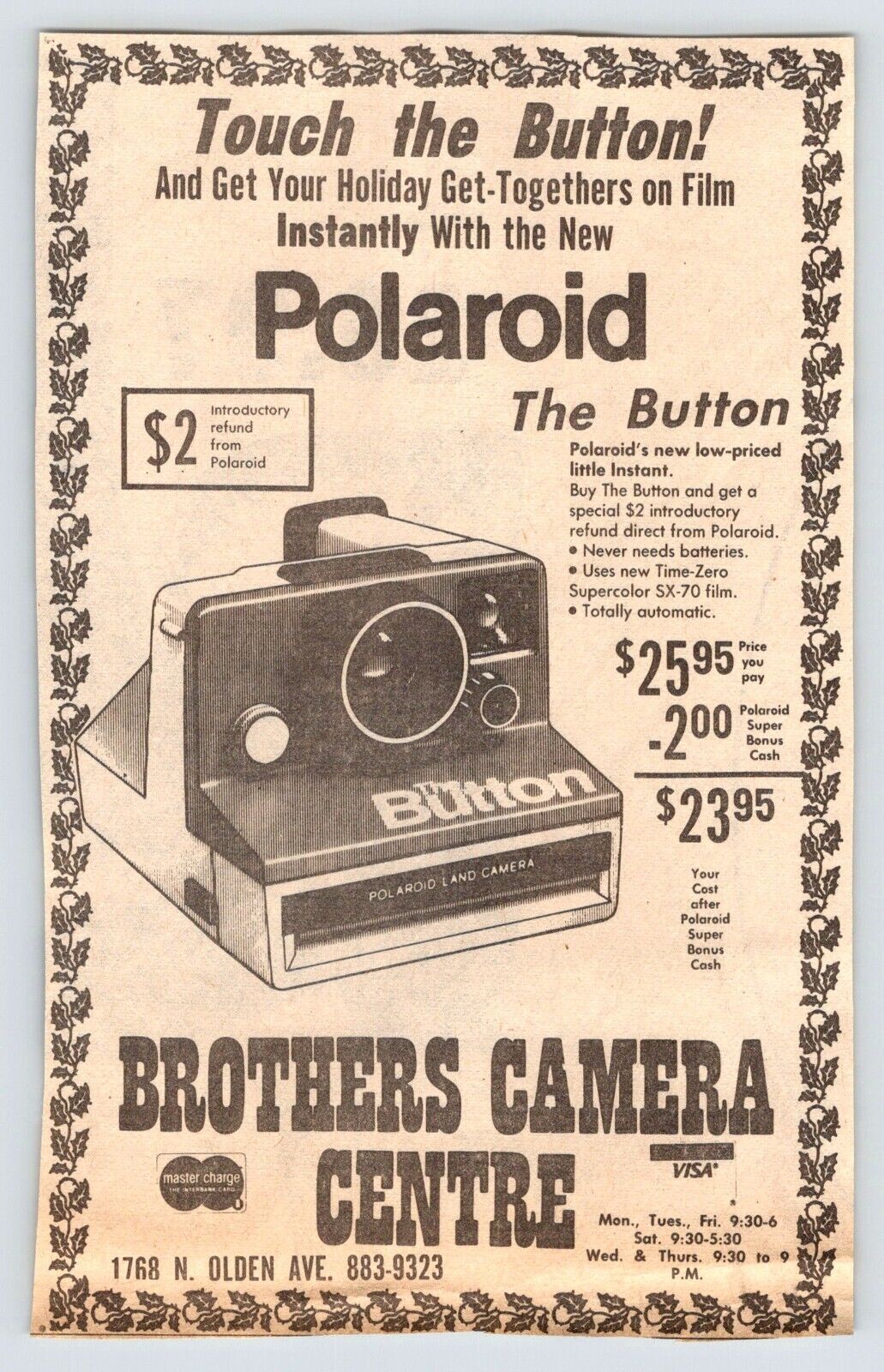The image features an old advertisement for a Polaroid camera, set against a white background. The central focus is a faded beige-yellow poster bordered by a chain of holly leaves. At the top of the poster, in bold lettering, it reads, "Touch the button and get your holiday get-togethers on film instantly with the new Polaroid." On the left side, the text promotes a special offer: "$2 introductory refund from Polaroid." On the right side, it showcases Polaroid's new low-priced instant camera, referred to as "The Button," available for $23.95 after the discount. Additional details highlight that the camera is totally automatic, never needs batteries, and uses the new Time Zero Supercolor SX-70 film. The advertisement also mentions that the camera is sold at Brothers Camera Center, which accepts Visa and MasterCard.